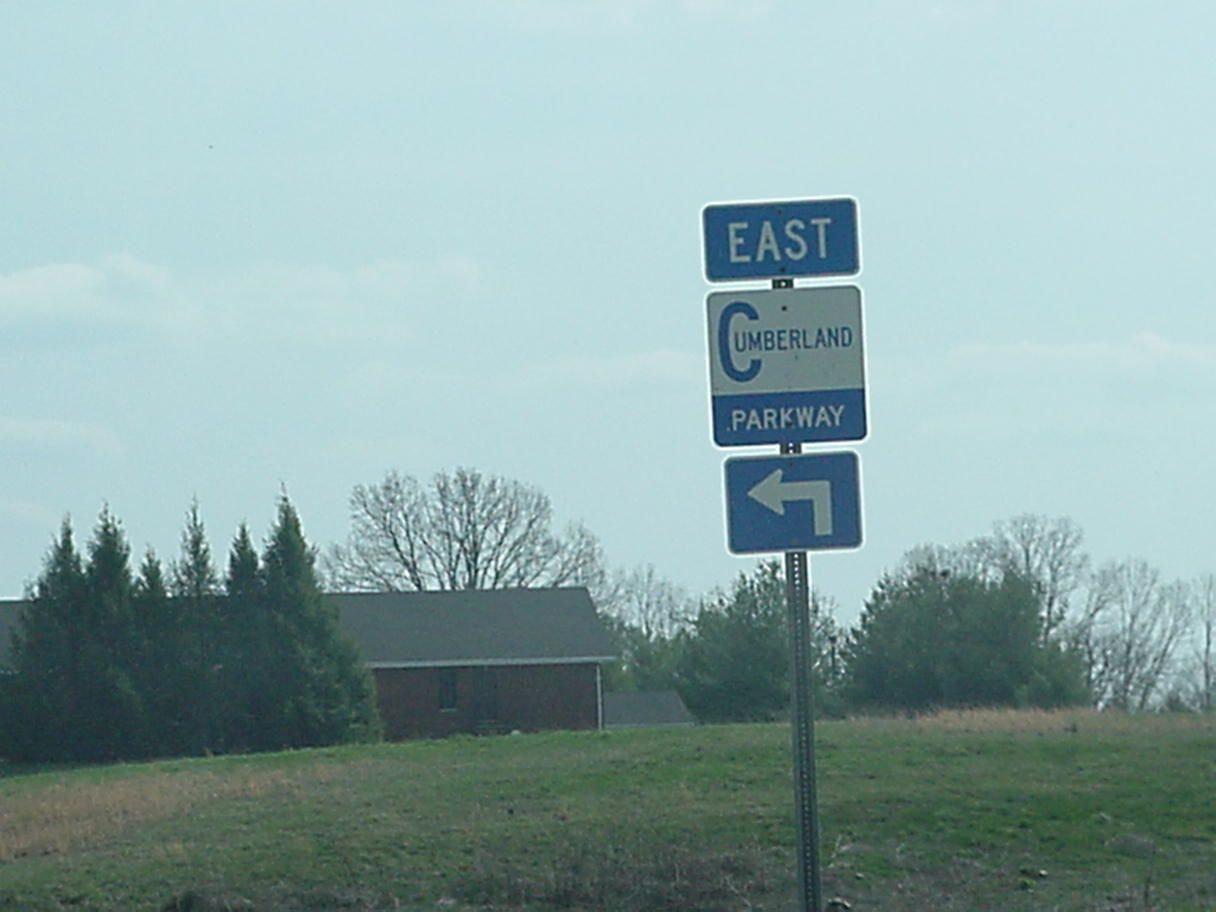The image depicts a roadside scene taken in the late afternoon with a clear, partly cloudy sky. Dominating the foreground is a multi-sign post positioned a few feet from a single-story red brick home. The top sign on the post features a blue background with white lettering that reads "East." Below it, another sign with a larger white top section and blue lower section displays the word "Cumberland" in blue letters on white, and "Parkway" in white letters on blue. The bottom sign shows a blue background with a left-pointing white arrow. 

The house, partially obscured by evergreen trees and situated towards the right middle of the image, adds a residential touch to the scene. The grassy area surrounding the house is well-maintained and features a mix of freshly cut grass and additional trees in the distance, including barren deciduous trees beyond the evergreens. The image's upper third displays the transition between the sky's grayish-blue hues and the descending sun, evoking a serene autumnal or early spring afternoon. Additionally, the rooftop of a nearby home is partially visible, hinting at a close-knit neighborhood setting.